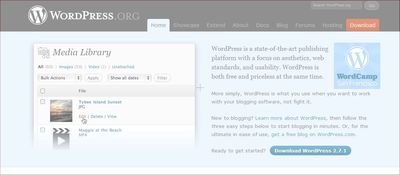The screenshot from the WordPress.org website features a prominent black navigation bar at the top, with links labeled "Home," "Blog," "Docs," and "About." Below this bar, there is a search function, followed by a main section set against a light blue background. This section includes a small image and a media library showcasing various content types, likely previews of WordPress's features. To the right of the media library, a text block describes WordPress as a state-of-the-art publishing platform. The text mentions the availability of version 2.7.3 for download. The top right corner displays a mention of "WordCamp," which likely refers to community-organized events for WordPress users. Overall, the website appears to mix both downloadable software offerings and cloud-based content management solutions.